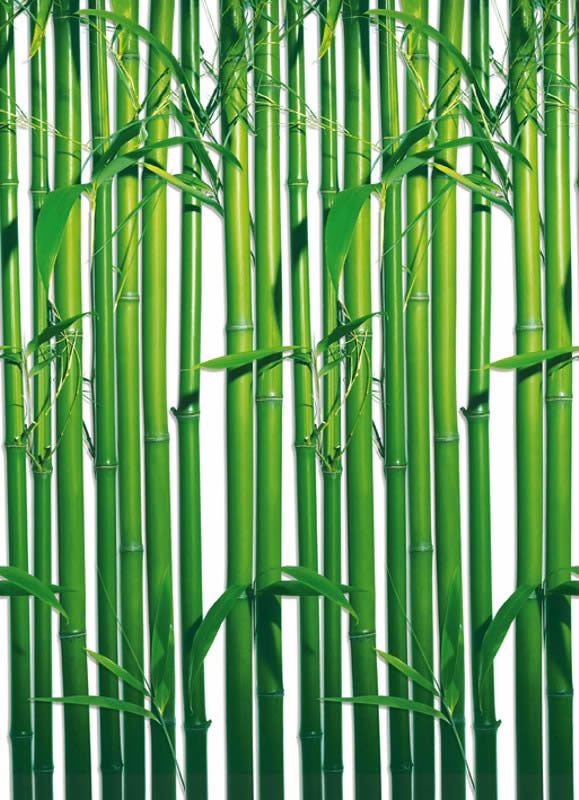The image appears to be a piece of digital or graphic art depicting 18 vertical stalks of bright green bamboo set against a white background. The bamboo stalks are tightly clustered, filling the frame from top to bottom, with small gaps where bits of the white background are visible. The stalks vary slightly in thickness and color, being darker at the ends and lighter in the middle, suggesting a light source slightly above and in front of the scene. Characteristic bamboo rings and slender leaves sprout from various points along the stalks, adding a natural, scraggly texture. There is no text or date stamp, and the entire image is in sharp focus, giving it a clean, almost design-like quality. This arrangement serves as a detailed demonstration of the plant's appearance, emphasizing the uniform yet varied nature of the bamboo.